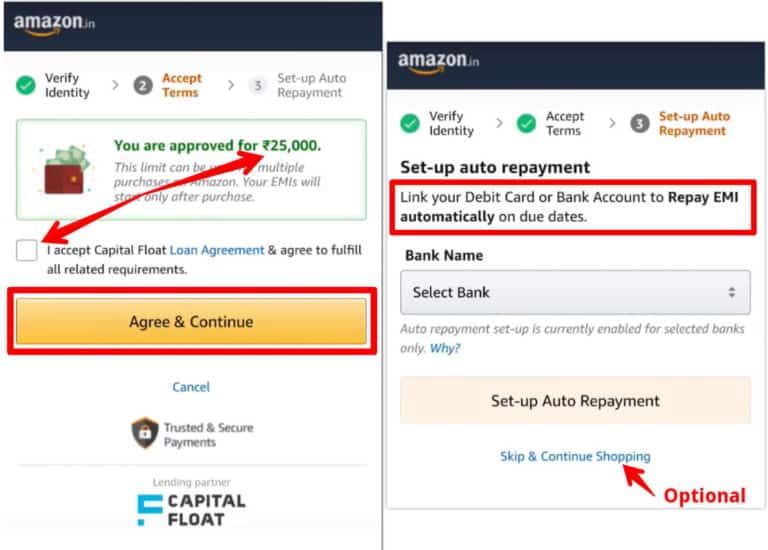**Caption:**

The image is divided into two sections, each displaying a webpage from Amazon, likely indicating a loan approval and setup process.

On the left side of the image:
- The topmost section features "Amazon.inc" with a yellow arrow underlined, set against a dark blue background.
- Below this, there are steps to be followed, listed on a white background:
  1. "Verify Identity" is checked with a green tick, indicating completion.
  2. "Accept Terms" is written in orange.
  3. "Set up Auto Repayment" follows next.
- Beneath the steps, there's a green text stating "You are approved for 25,000 rupees".
- A grey text is partially obscured by a red arrow, which points towards the amount and a checkbox that reads: "I accept Capital Float loan agreement and agree to fulfill all related requirements".
- Below this checkbox, there's an orange button with black text stating "Agree and Continue" outlined in red.
- Following this is a "Cancel" button in blue text.
- At the bottom, it mentions "Trusted and secure payment lending partner - F Capital Float", with "F" marked in blue.

On the right side of the image:
- The layout similarly starts with the Amazon webpage, where the first two steps are marked complete, indicated by green checks.
  1. "Verify Identity" – Completed.
  2. "Accept Terms" – Completed.
  3. "Set up Auto Repayment" is highlighted in orange and demands attention with text: "Set up auto repayment: Link your debit card or bank account to repay EMI automatically on due date".
- This step is encased in a red outline box.
- It further instructs to "Select Bank: Auto repayment setup is currently enabled for selected banks only".
- Below, there's an orange button labeled "Setup Auto Repayment".
- An alternative option provided is a "Skip and Continue Shopping" button in blue, with "Optional" written in red and linked to the button by a red arrow.

This detailed depiction showcases the user journey on Amazon's platform for setting up a loan repayment plan.